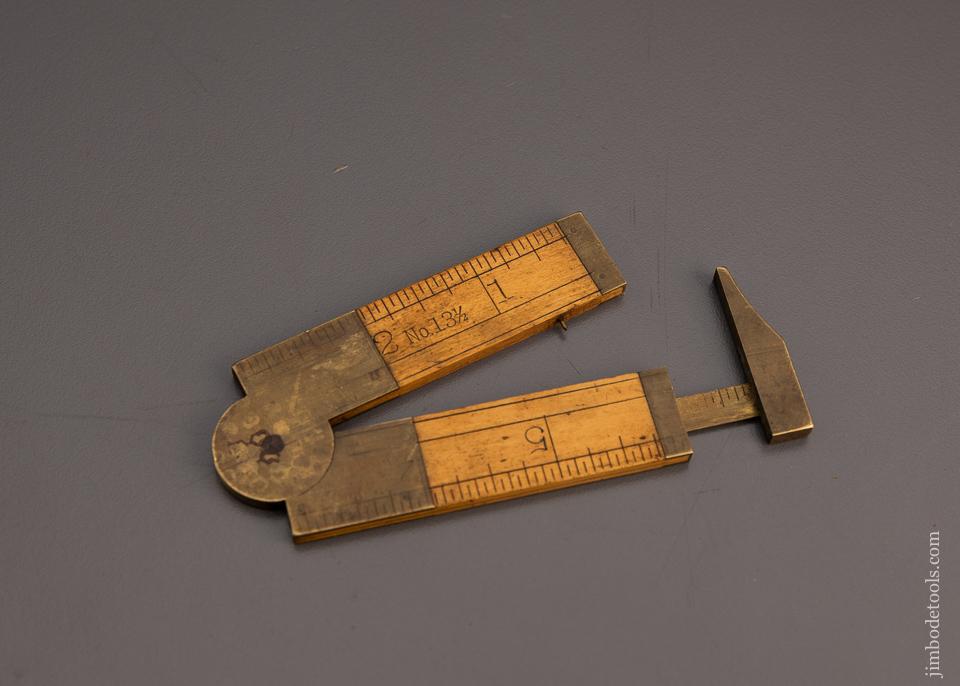The image showcases a vintage Stanley caliper ruler lying flat against a dark gray background. The tool is made of wood with metal components, possibly steel or bronze, giving it an antiquated appearance. Central to its design is a circular hinge or clasp, which connects two rectangular wooden arms that feature measurement markings in inches and centimeters. The ruler extends from 1 to beyond 6 inches when unfolded, with specific visible numbers such as 1 and 5. One end of the tool has a small, flat, hammer-like extension made of bronze. In the corner of the image, "jimbodetools.com" is faintly visible, adding to the vintage allure of this folding measuring instrument.